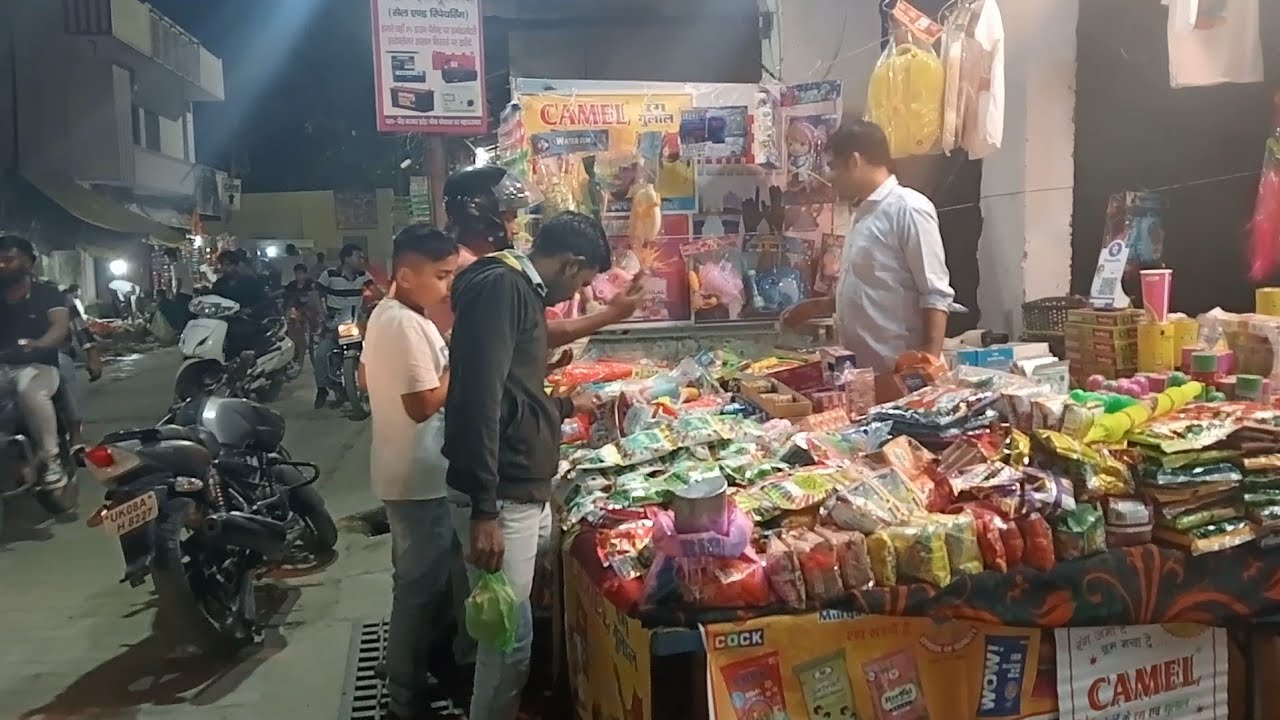This is a detailed night-time street scene photograph, likely set in an urban area of South or Southeast Asia. In the foreground, on the right side, there's a bustling market stall teeming with various goods, mostly wrapped in small, colorful plastic packages. Though hard to identify, these could include spices or other food products. The stall features a prominent camel poster, possibly for camel cigarettes, and another poster for a brand labeled "cock."

Attending the market stall is a vendor clad in a white button-down shirt with his sleeves rolled back, gazing to the right. In front of the stall, three individuals are intently surveying the products. One of them, a male in a green hoodie and faded jeans, holds a packet in his right hand. Another adult, slightly behind him, is partly obscured but wears a motorcycle helmet. Behind these two is a teenage boy with black hair in a white t-shirt and faded jeans. A streetlight illuminates the scene from the top-right corner, casting a glow on the gray concrete road. In the background to the left, a building stands amidst several motorbikes, some parked and some possibly being ridden, completing this vibrant urban tableau.